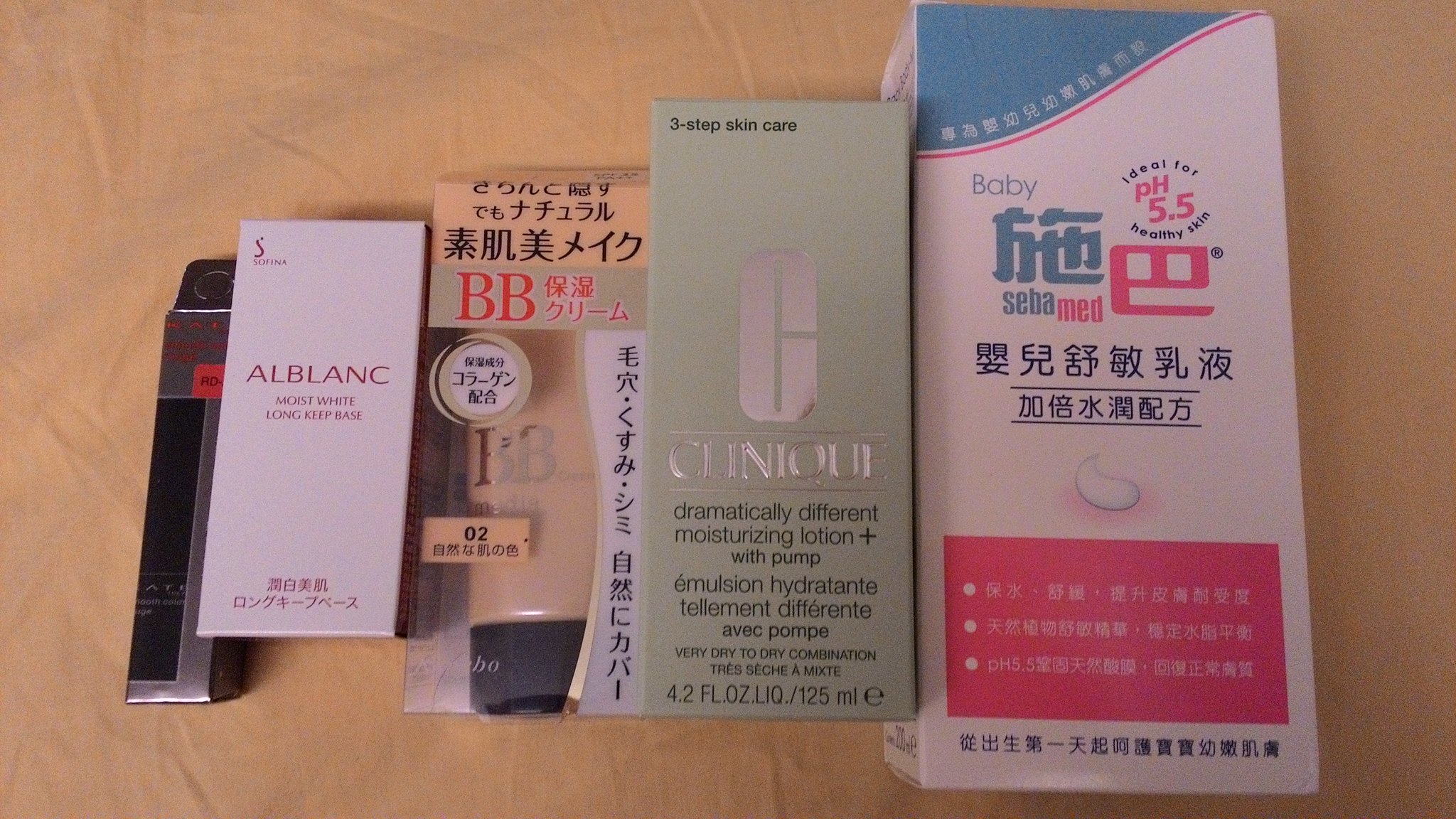The image displays a collection of five distinct beauty products, each with unique packaging and labels, placed on an orange-colored sheet. 

Starting from the left, the first product is a sleek silver and black box with red writing, featuring kanji characters, although the specific type of product is unclear. The second item is a white box labeled "Al Blanc Moist White Long Keep Base," and it also includes kanji characters at the bottom. The third product is housed in an orange-beige box with a transparent section revealing a beige-colored product inside marked with "BB" and featuring a black lid.

The fourth item is packaged in a muted green box with reflective silver writing that appears to spell "Clinique." The product name, "Dramatically Different Moisturizing Lotion Plus Whip Pump," is somewhat difficult to read due to the lighting. The final item on the right is the largest box, predominantly white with a blue top and red bottom, featuring an icon of cream in the center and various characters that are not easily legible. All the products rest on a sheet that has an orange hue.